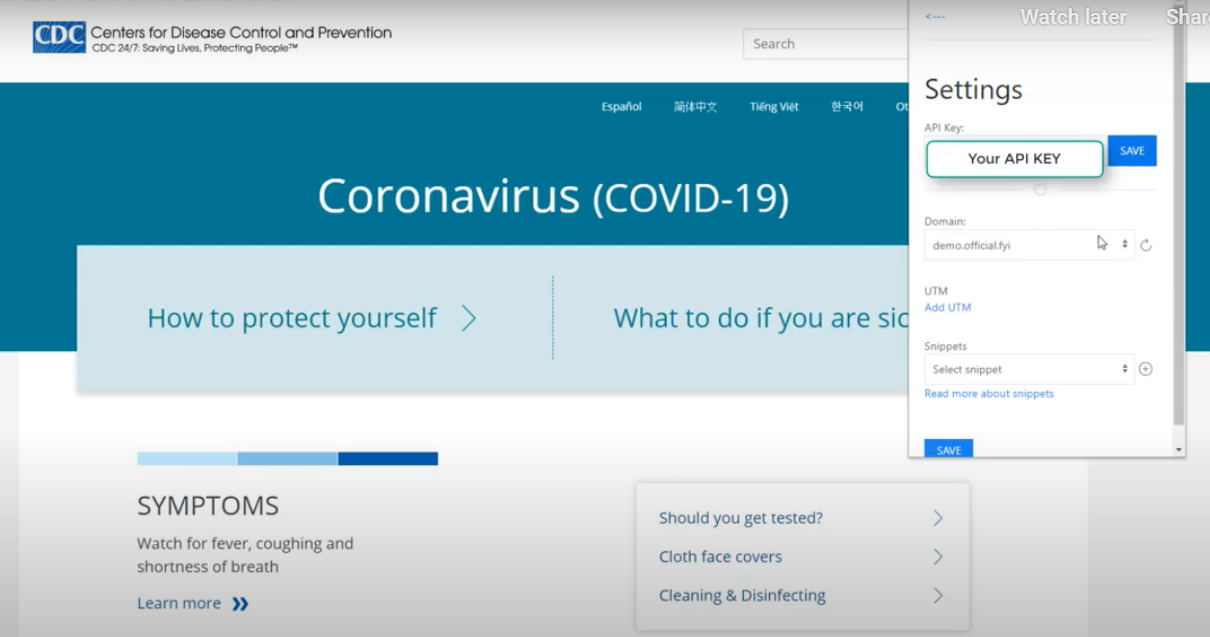The image features a CDC web page with a predominantly white, gray, and dark blue color scheme. 

1. **Top Left Corner:**
   - A dark blue rectangle with white text inside saying "CDC," encased within a dark gray bezel.
   - To the right of this is black text stating "Centers for Disease Control and Prevention."
   - Below it says "CDC" followed by "24/7: Saving Lives, Protecting People."

2. **Top Right Corner:**
   - A light blue-bordered rectangle with red text reading "Search."

3. **Main Section:**
   - A large rectangle with a gradient of dark blue and teal, featuring centered white text that reads "Coronavirus (COVID-19)."
   - Above this large rectangle are buttons for different languages, including Español (Spanish), a button resembling Chinese text, "Tagalong Viet" (Vietnamese), and another button which appears to be in Korean or Japanese, with one further button partially cut off.

4. **Right Sidebar:**
   - A vertical white rectangle containing black text that reads "Settings."
   - Instructions "Your API key is selected" pop out of this rectangle with a green border.
   - Next to it is a blue rectangle with white text saying "Save."

5. **Below Main Section:**
   - A light blue rectangle with blue text inside stating "How to protect yourself," accompanied by an arrow.
   - Following this are the words "What to do if you are SIC," with the text cutting off abruptly.

6. **Bottom of the Page:**
   - The word "Symptoms" is displayed at the very bottom.